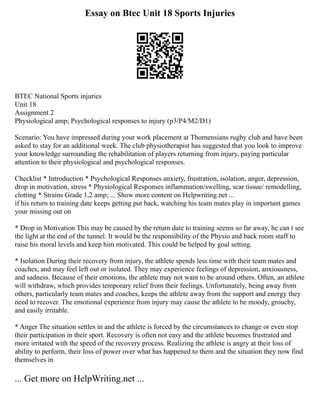The image depicts an essay titled "Essay on BTEC Unit 18 Sports Injuries," formatted in a portrait orientation on a white background with black text. At the top, in bold, is the essay title, followed by a centered QR code. Below the QR code, the essay is titled "BTEC National Sports Injuries Unit 18 Assignment 2: Psychological Responses to Injury." The opening scenario describes a student's extended work placement at Thor Missions Rugby Club, where they are advised by the club psychologist to enhance their understanding of player rehabilitation, focusing on both physiological and psychological responses. Detailed sections cover various psychological impacts of sports injuries, including a drop in motivation, isolation, and anger. Each of these sections explains how the athlete's return to training delays can affect their mental state, motivation, and feelings of isolation, along with the role of the backroom staff and psychotherapist in supporting the athlete through goal setting and emotional support. Physiological responses discussed include inflammation, swelling, scar tissue remodeling, and clotting related to grade 1 and 2 strains. At the bottom, in bold, is the website "getmorehelpwriting.net" for additional writing assistance.